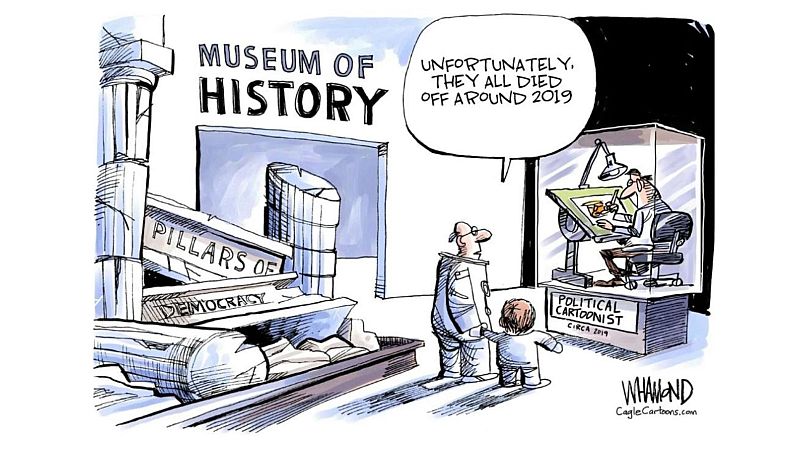This vibrant comic-style political cartoon by KegelCartoons.com captures a poignant and critical scene set within a dilapidated Museum of History. In the top left, a degrading concrete wall bears the words "Museum of History" in black letters, with the word "History" notably colored in. On the bottom left, the remnants of once-grand pillars, now fallen and labeled "Pillars of Democracy," are showcased behind a brown border, suggesting they were once displayed in pristine condition. Dominating the right half of the image, a father or grandfather holds a young child's hand as they examine a glass case labeled "Political Cartoonist, circa 2019." Inside the case, a cartoonist is seen diligently working at a drawing desk under a lamp. The elder figure has a speech bubble above his head that sadly reads, "Unfortunately, they all died off around 2019," addressing the extinction of political cartoonists. Both characters are inexplicably dressed in space suits, hinting at a distant future. The cartoon juxtaposes the decline of democratic pillars with the artistic commentary that once thrived, emphasizing how these crucial elements of society withered around 2019. The artist's name is discreetly placed in the bottom right corner, grounding the piece in its origin.